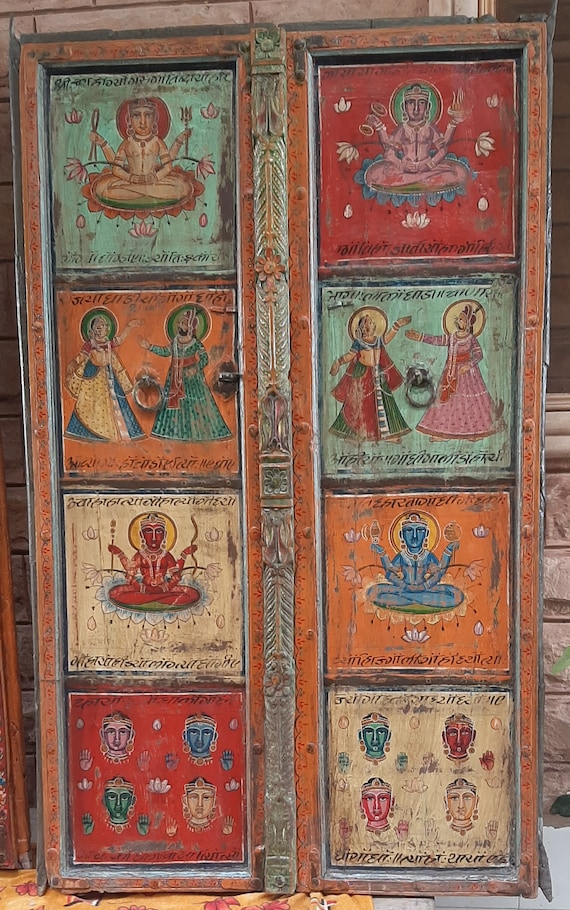The image depicts an antique, weathered wooden door or cabinet with a rectangular shape, showcasing eight intricately detailed square panels, four on each side. Each panel features vibrant, pastel crayon-like drawings depicting elements of Hindu art. The top two panels show an Indian God with utensils in hand, seated on a red floral pattern on an aqua background and a blue floral pattern on a red background respectively. The middle two panels display two figures in elaborate dresses—one with yellow and blue attire contrasted with green, and the other combination with red and green alongside blue and yellow, followed by pink and red dresses. The lower two panels once again feature the same Indian deity, this time on off-white and orange backgrounds. The final set of panels showcases four distinct heads against a red and an off-white background, evidencing the artwork's rich texture and aged appearance. The coordinated yet varied color palette, including turquoise, blue, orange, beige, red, and purple hues, enhances the detailed depiction of Hindu deities, creating a visually compelling artifact that speaks to its storied past.